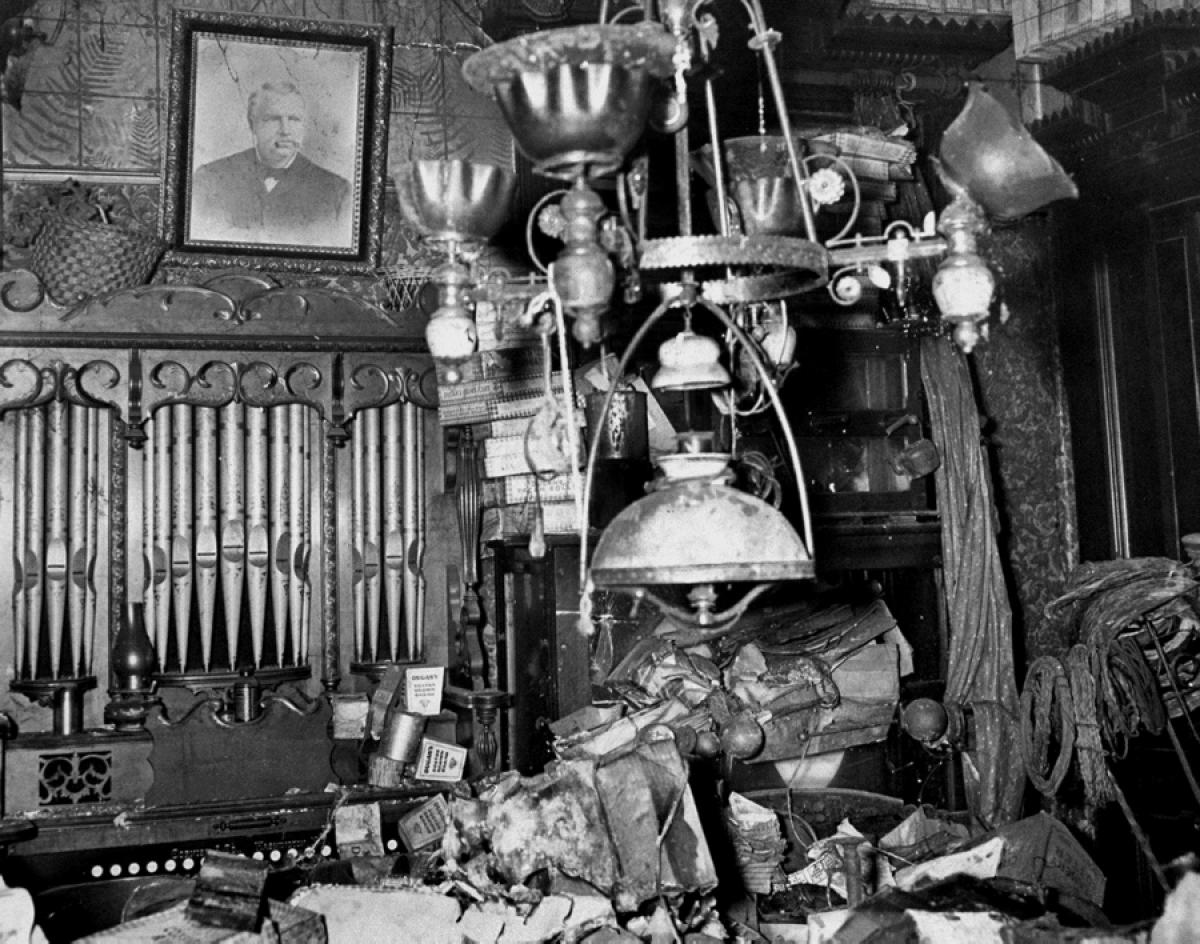This black and white photograph captures an abandoned and chaotic room, resembling a rundown church or possibly an old home. Dominating the left side of the image is a large organ with its pipes embedded in the wall, beneath which a collection of pull tabs can be seen. Above the organ, a framed black and white portrait of a man hangs, its glass cracked. In front of the organ, a table overflows with miscellaneous items, adding to the disorderly atmosphere.

In the foreground, a chandelier hangs low from the ceiling, appearing to be broken and missing some of its pieces. Surrounding this chandelier, the room is filled with a variety of scattered objects, including books and what may be scrolls, some piled haphazardly around the room. Toward the back, a tall hutch can be seen with items lined up inside of it, possibly including a vase and more books. The photograph evokes a sense of neglect and abandonment, with the disarray suggesting a past calamity, like a fire or general disuse over time. In the upper right corner, there is a hint of a towel or possibly a curtain rod with a curtain, adding to the overall sense of clutter and decay.